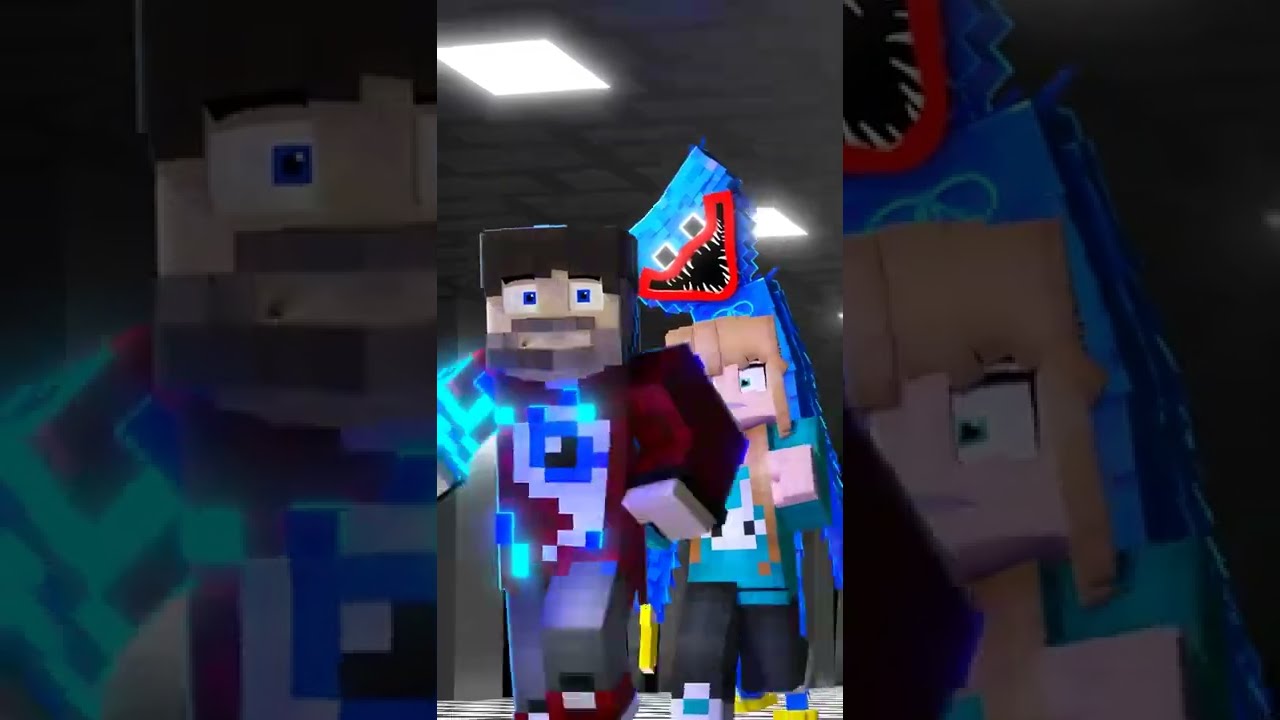The image is a screenshot, likely from a Minecraft animation or video game, depicted in a  portrait format, with the left and right sides of the image darkened and enlarged versions of the central scene. The scene features three pixelated, blocky characters reminiscent of Lego figures. The central male character has brown hair, a mustache, a beard, and blue eyes. He wears a red shirt with pixelated squares in green, red, blue, and white, along with silver pants. His outstretched red arm and blocky limbs add to his distinctive appearance. Directly behind him stands a female character with long, light brown to blonde hair, wearing a green shirt and black pants, exuding a cautious expression. Further back looms a menacing monster with a light blue body, jagged white teeth, thick red lips, and black eyes bordered in white, suggesting danger. The setting resembles a mine with white and gray ceiling lights, enhancing the adventurous theme. This detailed depiction hints at a narrative where the characters are sneaking away from the frightening monster, possibly as part of an animated adventure designed for a younger audience or as promotional content for the game.